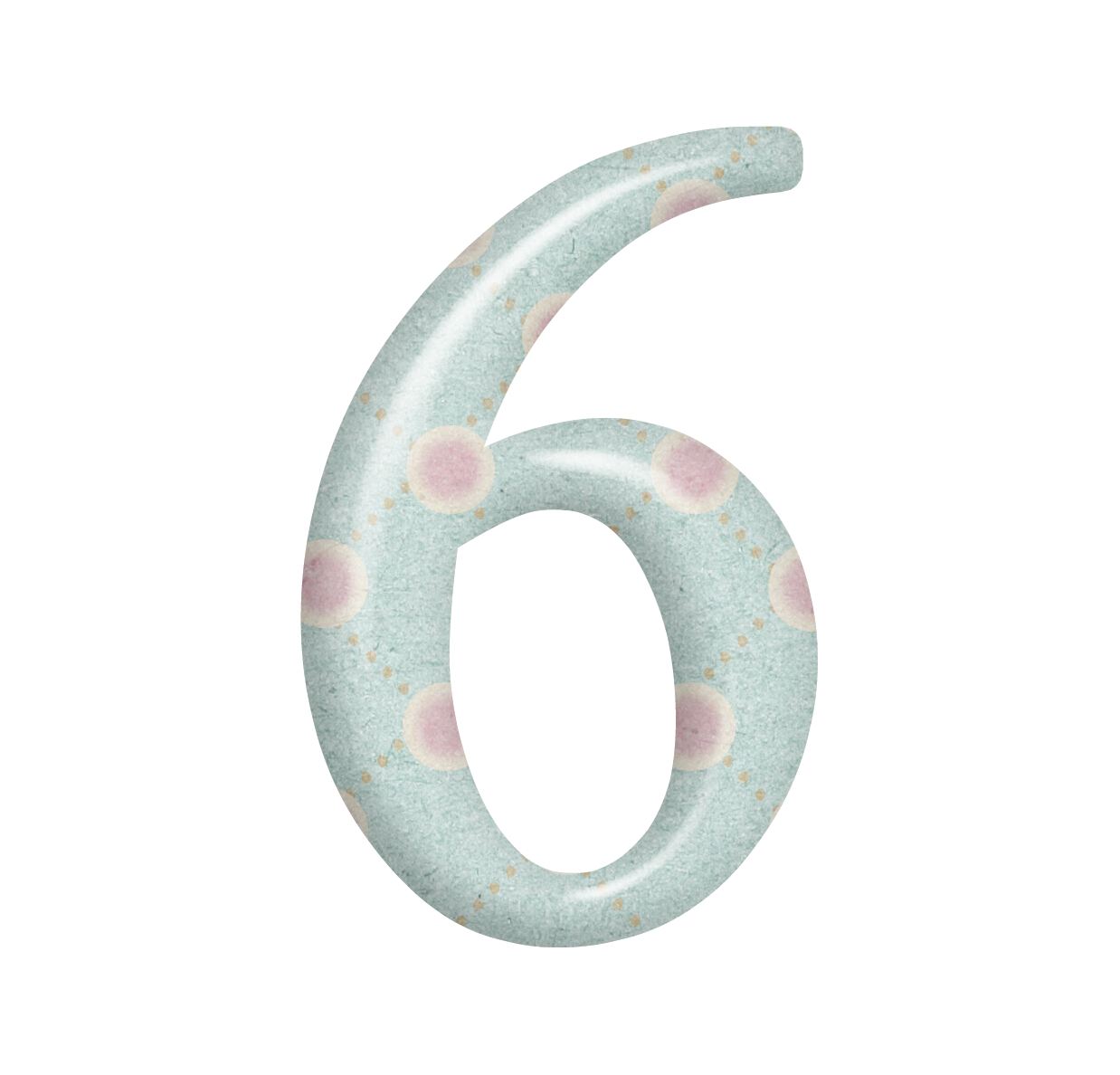The image depicts a bold, three-dimensional number 6 set against a white background. The number 6 has a smooth, turquoise blue or light teal hue, with a marble-like texture giving it a slightly reflective, almost soap-like or rubbery finish. The surface of the number 6 features a grid-like pattern of dots: large yellow circles with blurred red centers, connected by series of tiny pale yellow dots arranged in diamond shapes. The interplay of light on the number 6 accentuates its depth and three-dimensional quality, especially along the edges and curves. The overall appearance is somewhat cartoony, with the combination of vibrant colors and the whimsical dotted pattern enhancing its playful yet intricate design.